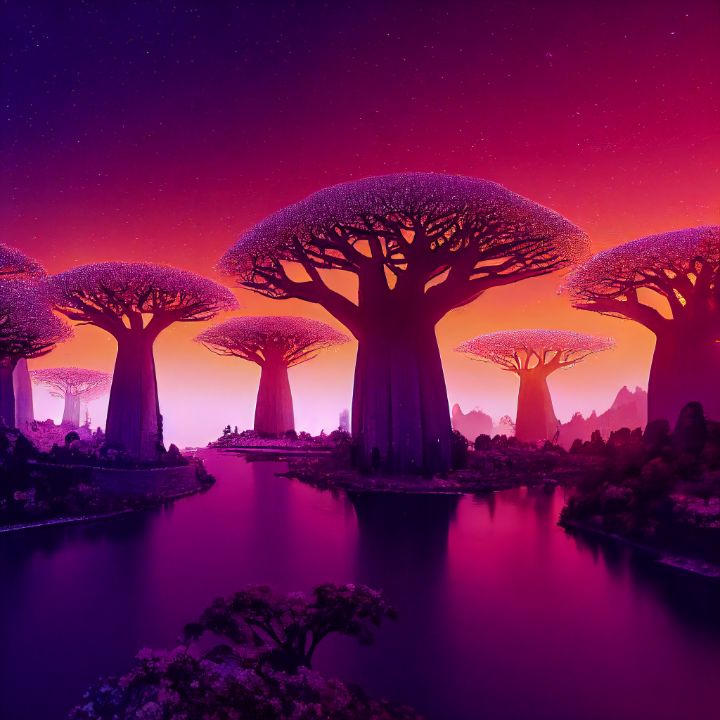In this digital image, we are transported to an otherworldly scene dominated by hues of dark purple and vivid orange. The foreground features very thick-trunked trees with round, massive bases. As they ascend, their trunks divide into sprawling branches that extend in all directions, culminating in purple leaves clustered at the tops. The largest tree stands prominently in the center, casting a black shadow that slices across the perfectly calm water below, reflecting the surrounding purple light.

On the bottom left, a bush with dark black and purple leaves juts upward, contrasting with the light. The background is populated by more trees, which, though identical in structure, differ in color. Trees on the left and in the back exhibit pink hues, while a tree on the right glows in orange. The foremost tree in the scene, stark in its very dark purple, stands out against this vibrant tapestry.

Above the trees, the sky transitions through a gradient of colors: it starts pale, almost white at the horizon, then shifts to lighter orange as it stretches downward, blending into pink and a darker purple at the top. The upper left corner of the sky is nearly black, intensifying the surreal atmosphere of this fantastical landscape.